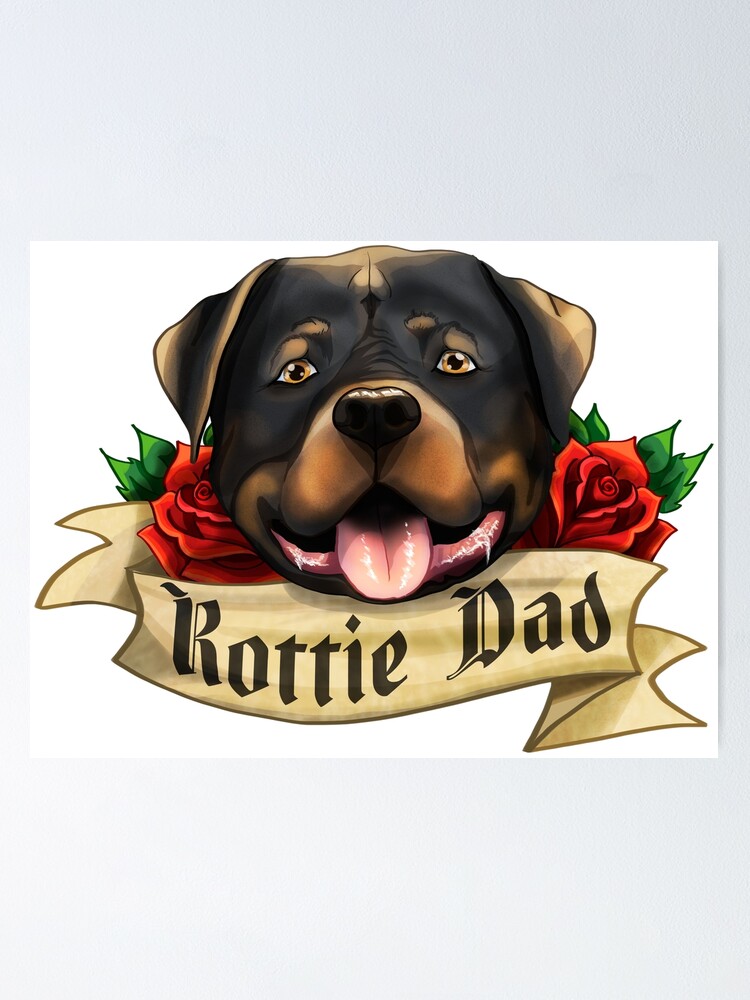The image is a detailed concept art for a tattoo featuring a Rottweiler. Centered in the white background, the dog is portrayed with a black and brown face, golden eyes, and floppy ears. Its mouth is open, revealing its tongue hanging out and a bit of drool dripping from the corners, giving the impression it's smiling. Framing the Rottweiler on both sides are vibrant red roses with lush green leaves. Below the dog, a tan ribbon banner flows with pointed edges, adorned with a script in a tattoo-style font that reads "Rottie Dad." The entire illustration is set against a light gray background, emphasizing the artwork's intricate details and design.